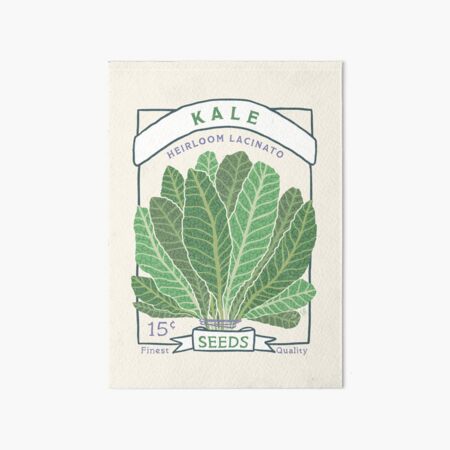This image features a drawing of a seed packet centered on a white or light gray background. The rectangular packet itself has a light beige, or off-white color, with a darker gray border that creates a vertical rectangle outline. A curved white banner across the top bears the word "KALE" in green letters. Below this banner, "HEIRLOOM LACINATO" is written in blue or purple text.

The main visual feature of the packet is an illustration of several kale leaves. These long, tapering leaves have a central vein with smaller veins branching out, and they point upwards and outwards from the middle of the illustration. The leaves range in color from a dark green to a lighter green. Toward the bottom of the packet, another white banner displays the word "SEEDS", with "15 cents" written in blue text just below the left side of the leaves. The bottom of the packet is further adorned with the words "FINEST" and "QUALITY" on the left and right sides respectively.

Overall, the design and text create a detailed, visually appealing presentation for a packet of heirloom Lacinato kale seeds, emphasizing both the quality and affordability of the seeds.